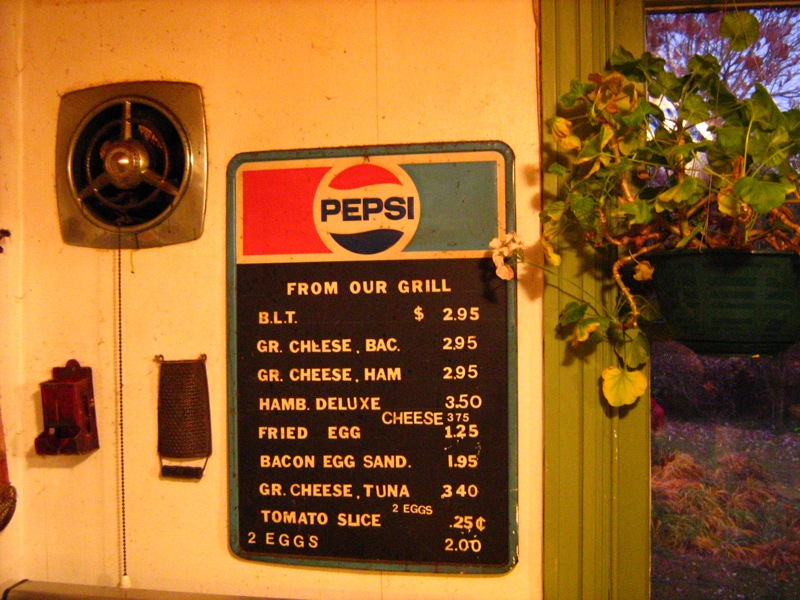This image features a vintage Pepsi Cola sign from what appears to be the late 60s to 70s, though it may have been photographed more recently using film. The classic Pepsi logo crowns the sign, below which a black background showcases a list of menu items in white text. The offerings include a BLT for $2.95, a grilled cheese bacon for $2.95, a grilled cheese ham for $2.95, a hamburger deluxe priced at $3.50, a fried egg for $1.25, a grilled cheese tuna for $3.50, tomato sauce for $0.25, and two eggs for $2.00. These prices suggest the sign likely dates back to around 1997. To the right of the sign hangs a plant that shows signs of neglect. On the left, the wall displays an assortment of old, small silver items. This nostalgic setting evokes a sense of a bygone era, further accentuated by the condition and style of the items surrounding the prominent and well-preserved Pepsi sign.